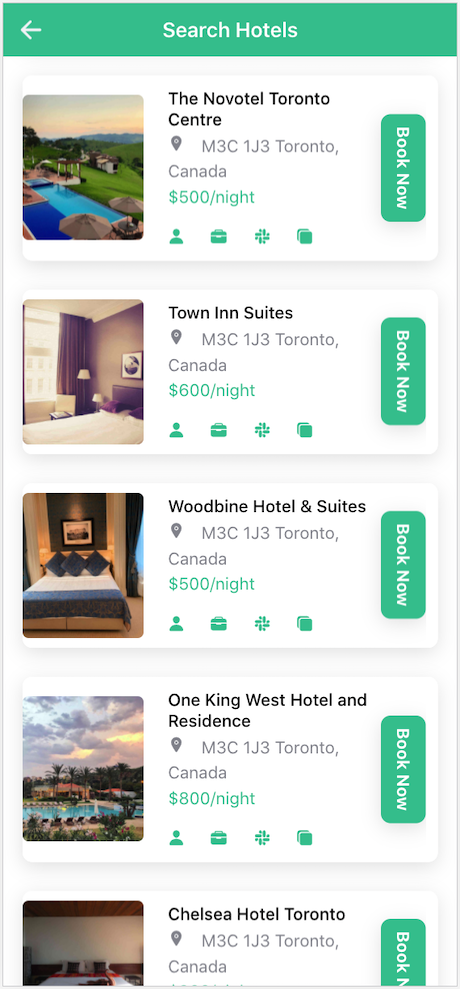The image depicts a smartphone screen displaying a selection of hotel options in Toronto, Canada. At the top of the screen, there's a greenish rectangle featuring an arrow pointing to the left. The first listing is for the Novotel Toronto Center, priced at $500 per night, with a "Book Now" button prominently displayed. 

Below this, the Town and Suites hotel is listed at $600 per night, also in Toronto, with a "Book Now" button. Each hotel listing includes a small image on the left and a row of green icons at the bottom, depicting a silhouette of a person, a chest, a plus sign, and squares.

Scrolling further down, Woodbine Hotel and Suites in Toronto are shown at $500 per night, accompanied by a similar "Book Now" button. The One King West Hotel and Residence is next, listed at $800 per night, again with a "Book Now" button.

The final listing is for the Chelsea Hotel in Toronto. However, the price is partially cut off, displaying only "book" and a partial "N," indicating a "Book Now" button. All entries display consistent formatting with images and booking options.